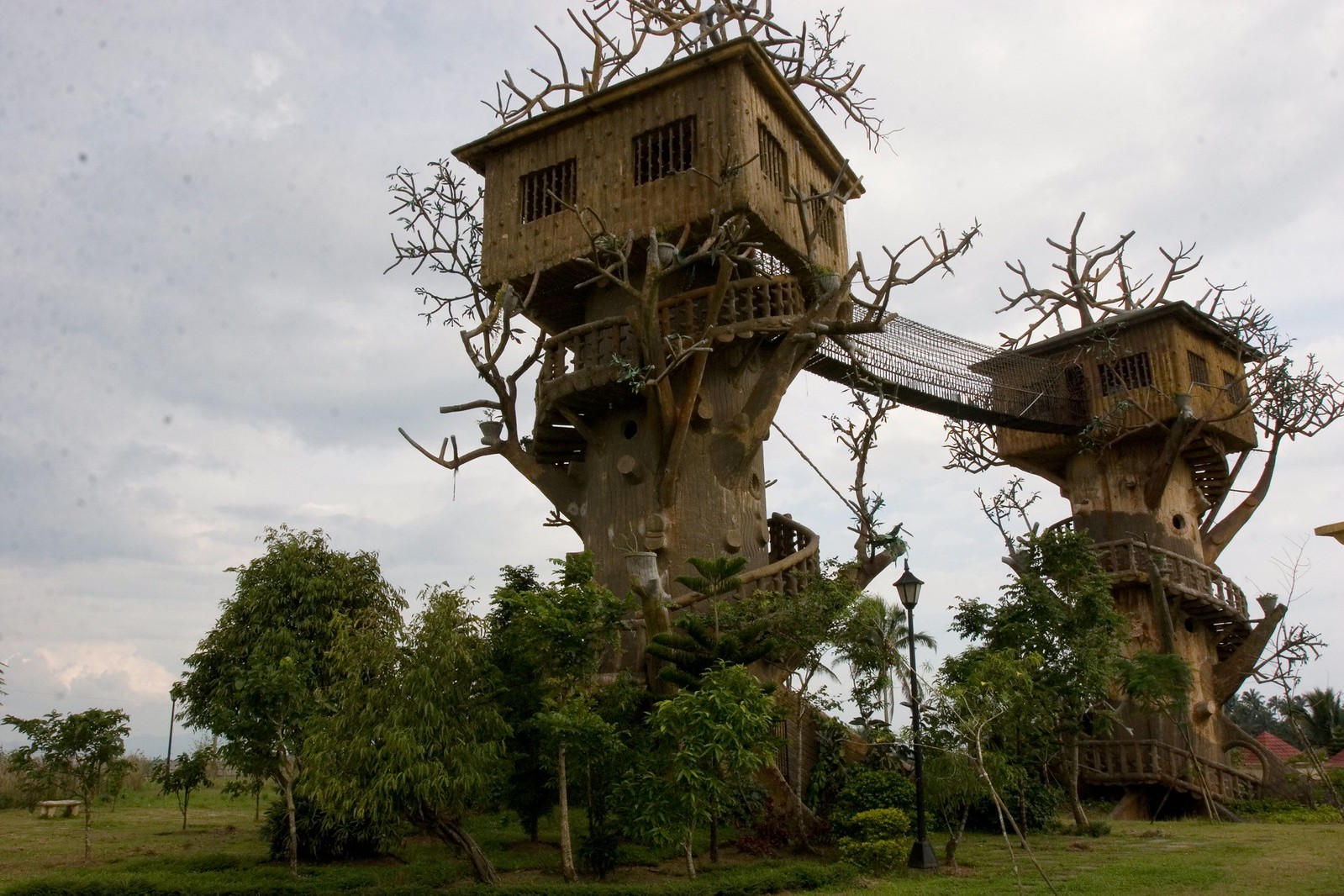In this horizontal outdoor image, featuring an overcast sky with wispy clouds, two fantasy-inspired treehouses are prominently displayed, evoking a scene straight out of a magical movie. These man-made treehouses are mounted atop thick, cylindrical, barren tree trunks, giving an impression of artificiality. The verdant surroundings are a mix of lush green trees, small leafy trees, and palm trees, with grass that varies from light green to dark green and brown patches.

Each treehouse, constructed from dark brown plank wood, features flat roofs and two rectangular windows on each side, which are fitted with bars for added authenticity. Short artificial limbs and additional branches protrude from both the trunks and the tops of the treehouses, enhancing their fantastical look. A wooden staircase spirals gracefully around each trunk, connecting the ground to the elevated treehouses.

At the top, a high-netted suspension bridge with safety nets on both sides links the two treehouses, creating an adventurous pathway between them. Additional elements include a vintage lamppost positioned at the base of the treehouse, casting a soft glow over the scene, and glimpses of red-roofed houses in the background, adding to the charm and detail of this whimsical setting.